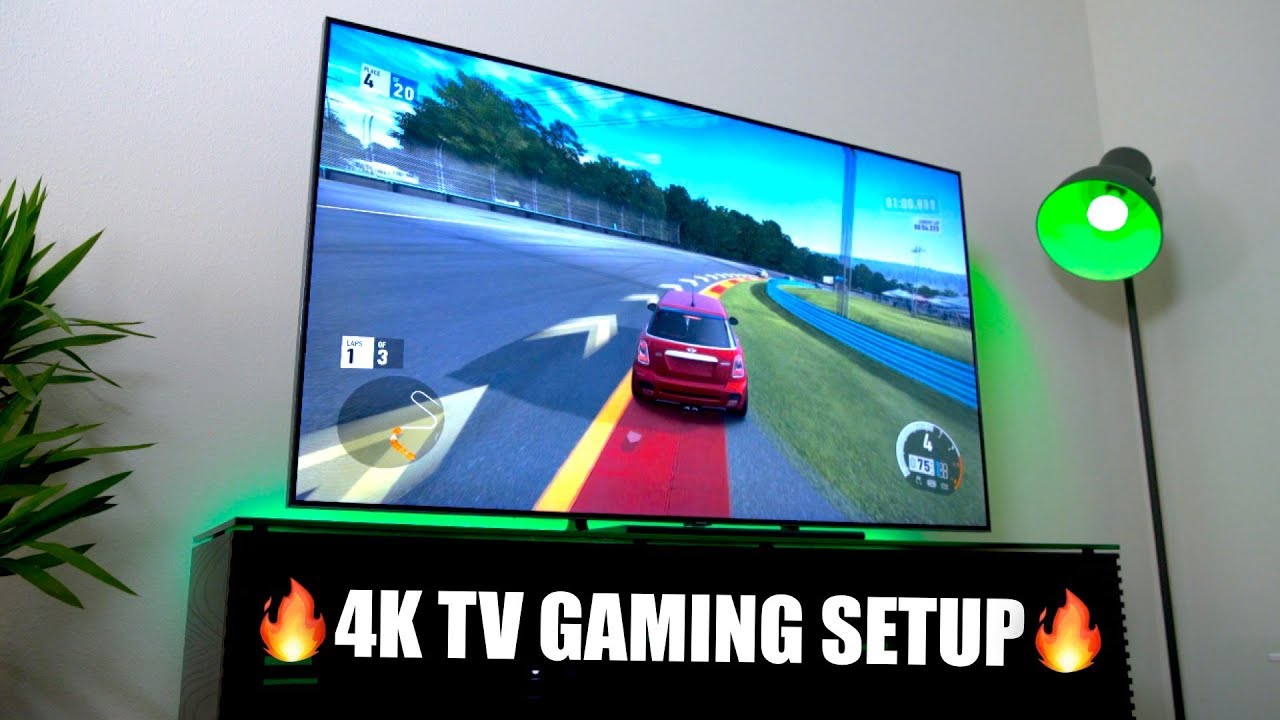The indoor photograph showcases a sophisticated gaming setup against a gray, cornered wall. Dominating the scene is a flat-screen TV mounted on a black cabinet. The TV screen displays a vivid video game scene featuring a blue sky, trees, a fence, and a racetrack with a small car veering off-course. Beneath the TV, white text reads "4K TV Gaming Setup," flanked by fiery flame emojis. A tall, black pole lamp on the right emits a greenish light, casting a subtle glow across the room. On the far left, partially visible, are the long leaves of a plant, adding a touch of greenery to the modern gaming space.